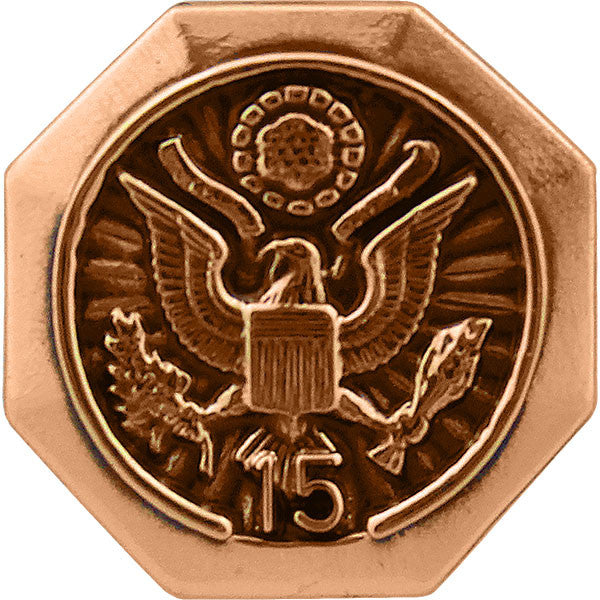The image shows a close-up view of a single object, a detailed and shiny metal item, likely a coin or a plaque, set against a solid white background. The object, which appears to be a commemorative or antique piece, takes up most of the photo and is positioned centrally. The coin or plaque features an intricate design: an eagle with spread wings and a shield over its body. The eagle's legs are extended, each grasping what looks like two plants. The whole design is encased in a copper-colored border shaped like an octagon but giving a substantial, sturdy appearance. Surrounding these details is a circular border, within which the number "15" is prominently displayed at the bottom. The dominant colors of the object are tan, dark brown, and light brown, adding to its vintage, possibly military or historical aesthetic. There is no text beyond the number "15," suggesting that this might be a symbolic or thematic piece, possibly linked to a museum exhibit or an old currency system.